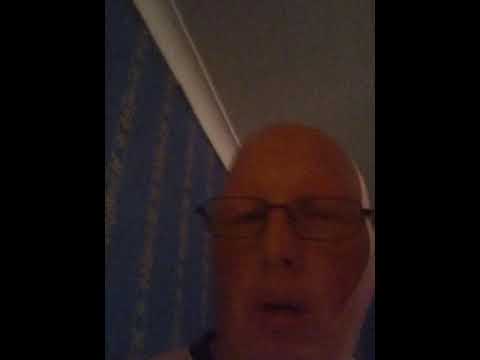This is a slightly blurry and dark image of a man’s face, likely taken during a FaceTime, Skype, or Zoom call. The man appears to be in his 50s or 60s with a bald head and wearing glasses. His face occupies the lower right quadrant of the image, with his mouth slightly open as if he is in the middle of saying something. He has a reddish hue to his complexion. Just the top of his t-shirt collar and one shoulder are visible. Behind him, the wall to his left features blue wallpaper adorned with silver stripes, and above it, white trim separates the wall from a gray ceiling. Additionally, there are vertical black borders on the left and right sides of the photo, and a light source from the right side illuminates part of his face.